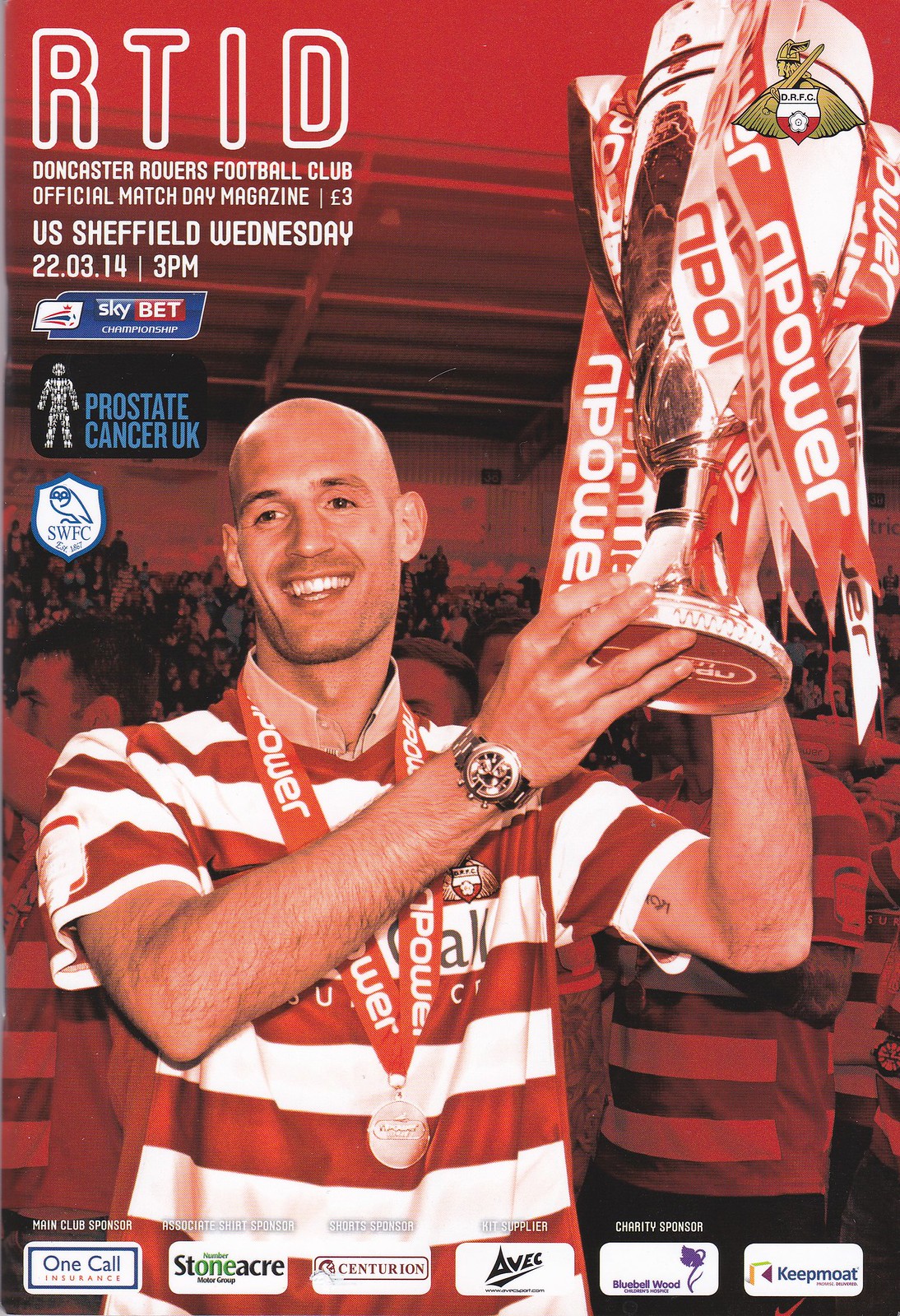The cover of the magazine features a dynamically centered image of a jubilant soccer player from Doncaster Rovers Football Club, proudly displaying a gleaming silver trophy adorned with red and white ribbons. He sports the team's signature red and white striped jersey and has a thick red ribbon around his neck that holds a round, silver medallion. A black-banded metallic wristwatch is visible on his right wrist. Behind him, the background is a vibrant depiction of stadium seating filled with spectators, tinted with red hues, enhancing the celebratory atmosphere. At the top, large white text reads "RTID," with smaller text below announcing "Doncaster Rovers Football Club Official Matchday Magazine." Additional details include "3lb U.S. Sheffield Wednesday 2203 14 3pm." Below this header, there is a rectangular "Sky Bet" logo and another sponsorship logo. Six more sponsors, featuring colors like blue, black, green, and purple, are aligned across the bottom of the cover, adding to the visual impact of this matchday program for an English soccer team.